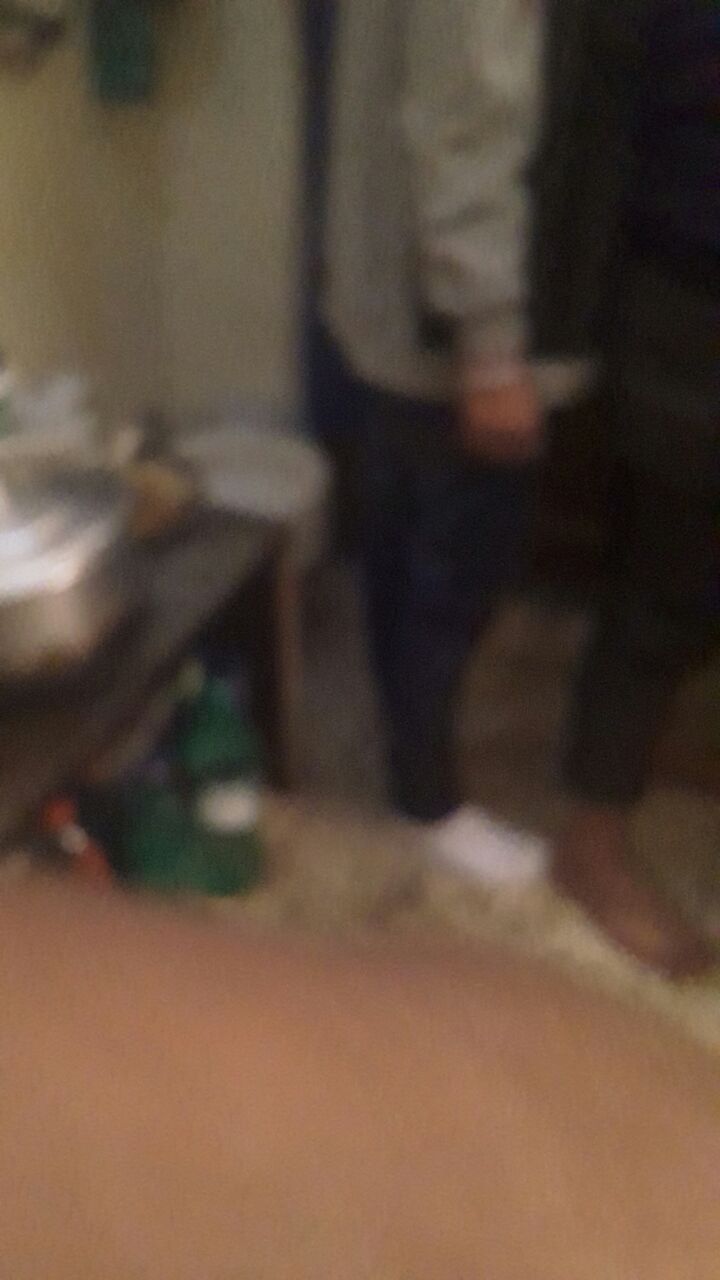In a horizontal, blurry photograph, two individuals stand side by side. The person on the left is dressed in long black pants, white shoes, and a long-sleeved gray sweatshirt adorned with a black rectangle across the front. The individual to the right is barefoot, clad in long black pants and a black shirt. They appear to be engaged in putting on a brown boot, with the left foot sporting a white sock. Behind them stands a dark chocolate brown table supported by lighter brown legs. Atop the table sits a silver pot with a rust-stained lid. The table also holds various indistinguishable items due to the blur, and green bottles with white packaging are partially visible beneath it. The room features a light tan and dark brown carpet and walls painted a white cream color, with a small cylindrical white object resembling a trash can situated against the wall. Additional objects, including a green rectangular item, hang in the left corner of the room.